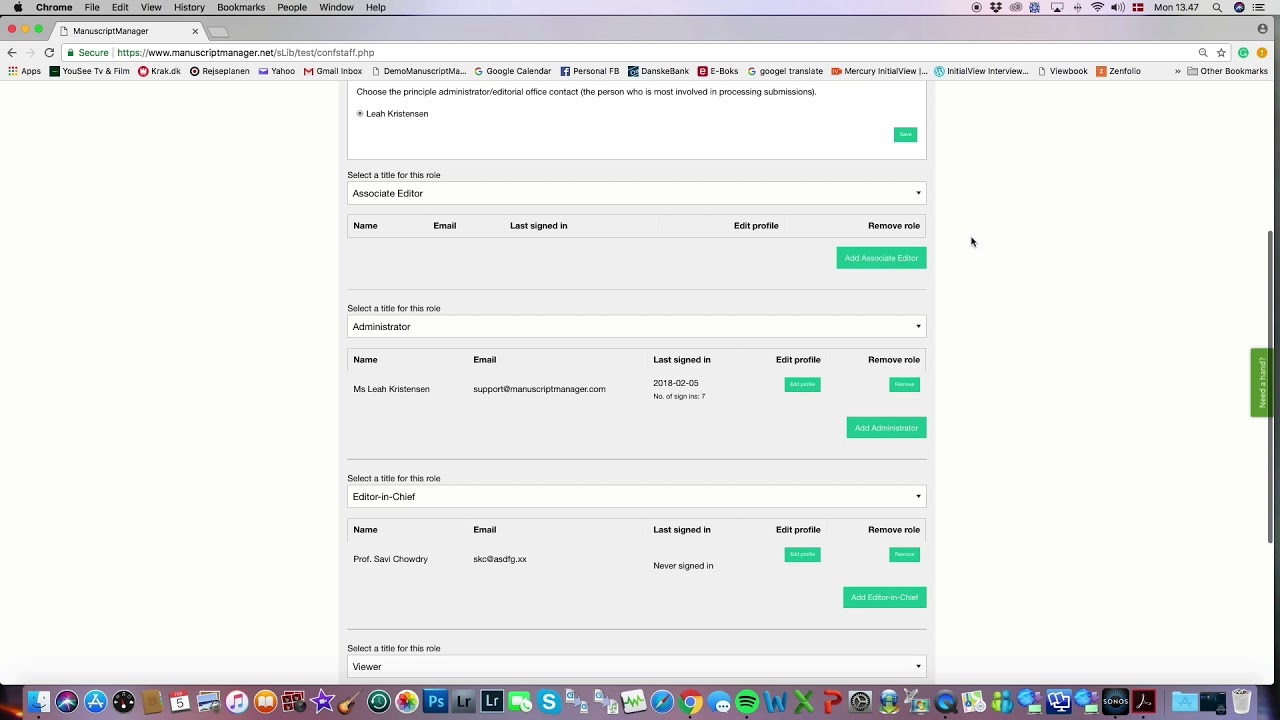This screenshot captures a cluttered desktop interface. At the top of the screen, the Apple menu bar is visible, featuring the Apple logo—a stylized apple with a bite out of it—on the far left. This is followed by drop-down menus labeled File, Edit, View, History, Bookmarks, People, Window, and Help. In the far right corner of the menu bar, there are several icons indicating sound control, internet connection status, a search bar, and the current date and time.

Below the menu bar is the browser's tab interface. The left corner is dominated by the typical red, yellow, and green close, minimize, and maximize buttons, respectively. Adjacent to these buttons, the title "Manuscript Manager" is displayed. The active tab, titled "Manuscript Manager," reveals the secure website address ManuscriptManager.net in the web address bar, denoted by a padlock icon as a sign of security. 

Pinned beneath the web address bar are several shortcut buttons for various applications, including email and personal Facebook, among others. The main window of the Manuscript Manager application is open, displaying sections for name, email, profile, associate editor status, sign-ins, and emails. These elements are organized into horizontal rectangles that stack vertically. Blue action buttons are interspersed within these sections.

The desktop's bottom taskbar is completely filled with application icons, including Spotify and Chrome, among many others. The assortment of icons creates a cluttered appearance across the bottom edge of the screen.